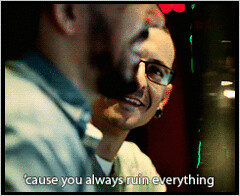This small, almost square-shaped picture with a black border captures a candid moment between two men. The man in the foreground is partially visible from his nose down to his shoulders, sporting a full brown beard and mustache, and wearing a gray or light blue collared button-down shirt. His face is somewhat blurry, suggesting he was moving or that the camera was slightly out of focus. To his left, the other man, who appears to be bald or sparsely haired on top, is more in focus. This man is wearing glasses and smiling broadly, showing his teeth. He seems amused, possibly engaged in a friendly conversation with the man in front of him. A light source is barely visible on the right middle edge of the photo, illuminating part of their faces but not revealing much of the dark background. At the bottom of this snapshot, white text reads, "'Cause you always ruin everything." The overall scene hints at a light-hearted interaction, perhaps in a casual or social setting.